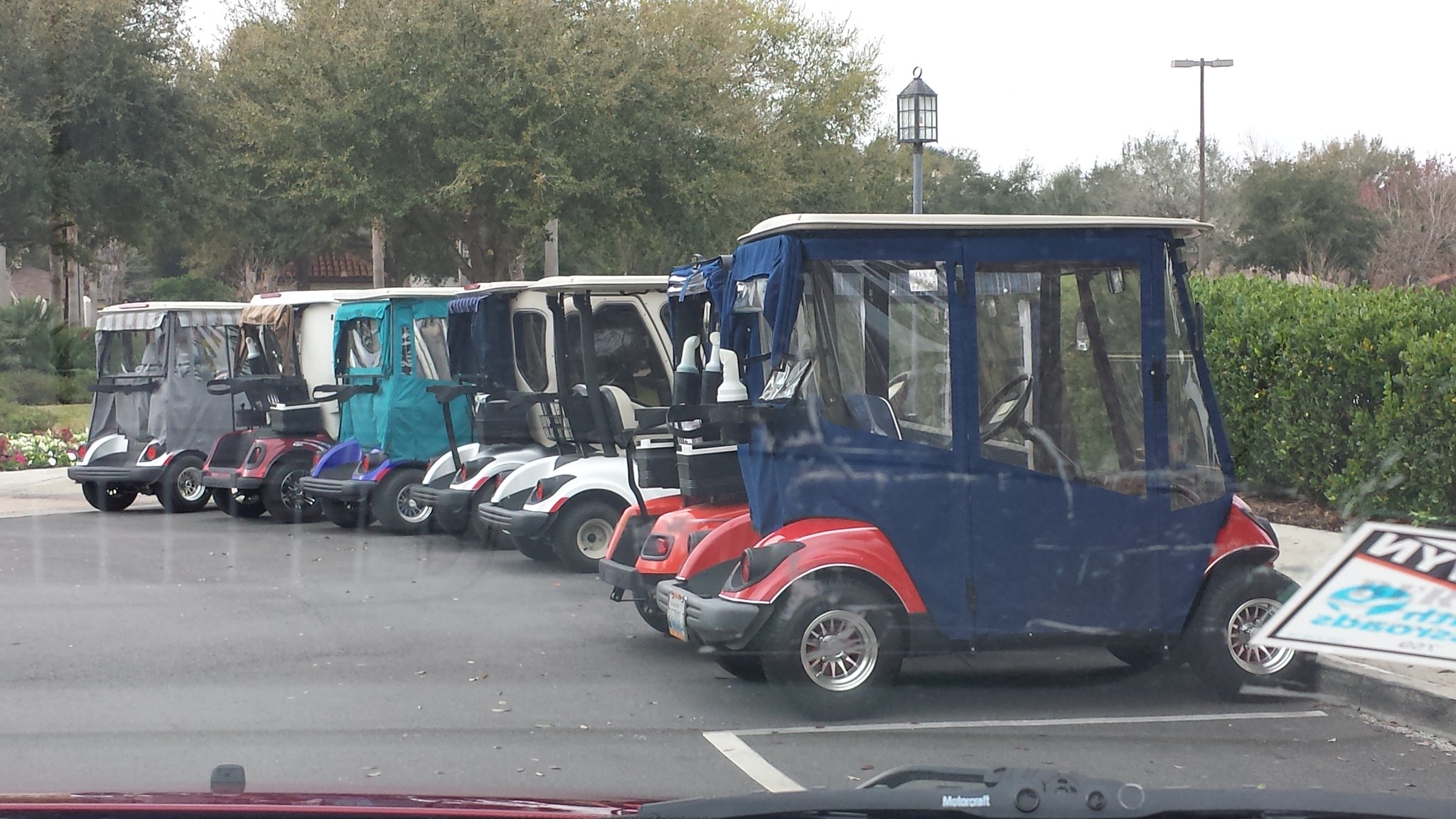The image is a detailed, realistic photograph taken outdoors during the day in a large parking lot. Centered in the parking lot are a line of small vehicles that appear to be golf carts, each covered with protective rain gear. There are 10 golf carts in total, each fitted with a little steering wheel. The carts are arranged in a neat row, including two red ones, three white ones, a blue one with red accents, a turquoise one, a white one with burgundy accents, a grey one with a grey cover, and others with blue, green, and black covers. Both red and purple carts are mentioned. In the foreground, from a vehicle with a windshield wiper, labeled "Motorcraft," the scene unfolds. Behind the carts, tall green trees dominate the left side of the background while shorter hedges are on the right. A bed of flowers composed of red, white, and yellow bursts of color adds a touch of nature. Protruding leaves of some trees show diverse hues, including purple and orangish-brown. The bright white sky above suggests a cloudy day, and a partially visible sign, possibly damaged, featuring the letters "Y N" and various colors, adds to the ambiance. There are no people in the photograph.